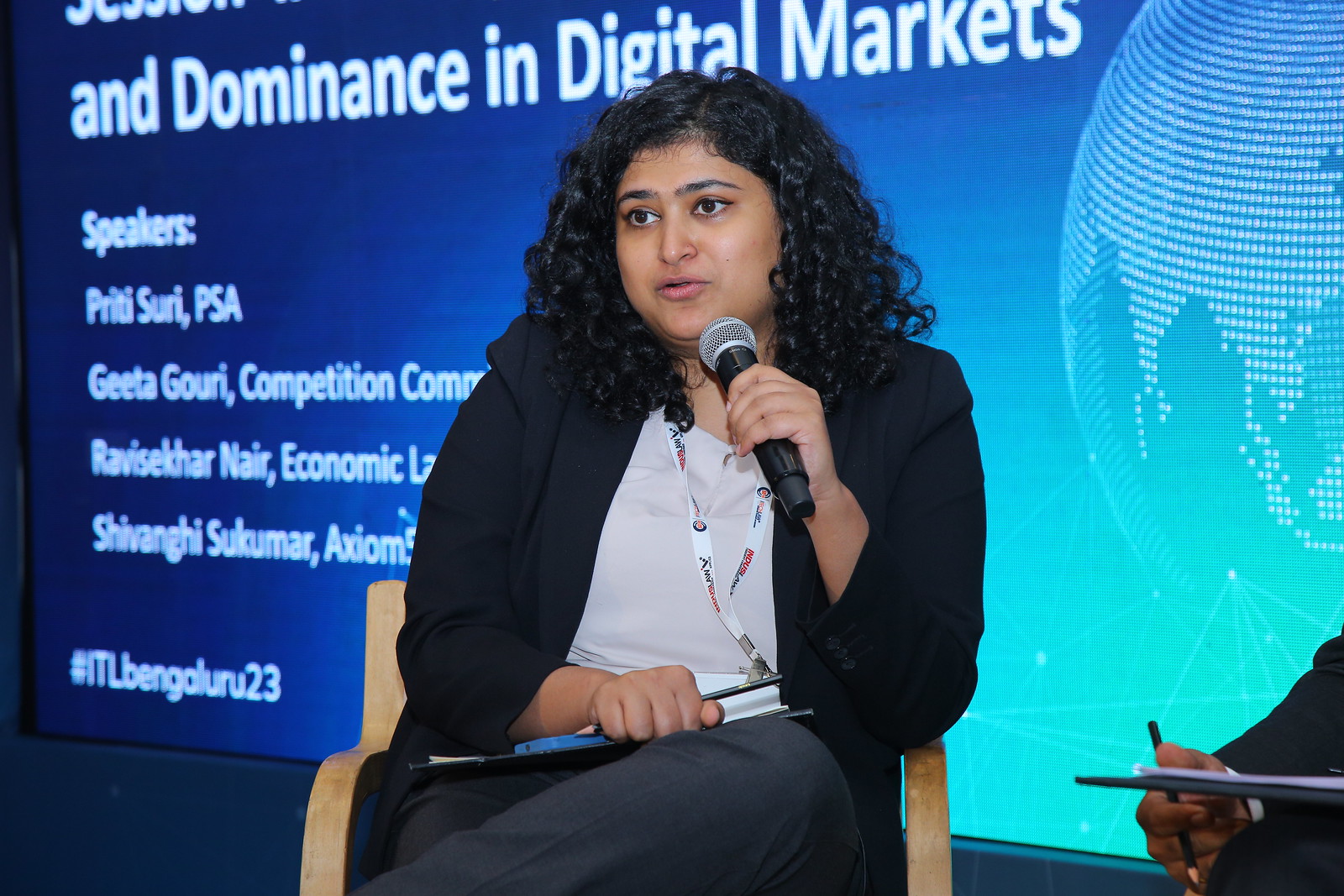In this photo, taken at a conference, the focus is on a female presenter of apparent Indian descent with dark black curly hair. She is wearing a black blazer over a white top and gray pants, with a lanyard around her neck. Seated in what appears to be a high-backed chair, she is holding a microphone and speaking, her eyes directed towards the audience. She also holds writing material in one hand. In the background, there is a gradient blue presentation screen featuring a globe graphic. The readable text on the screen includes "End Dominance in Digital Markets" and lists speakers: 'Priti Suri, PSA,' 'Greta Guri, Competition and Communication,' 'Ravi Sekar Nair, Economics,' and 'Shivangi Sukmar.' The screen also features the hashtag '#ITLBengaluru23.'